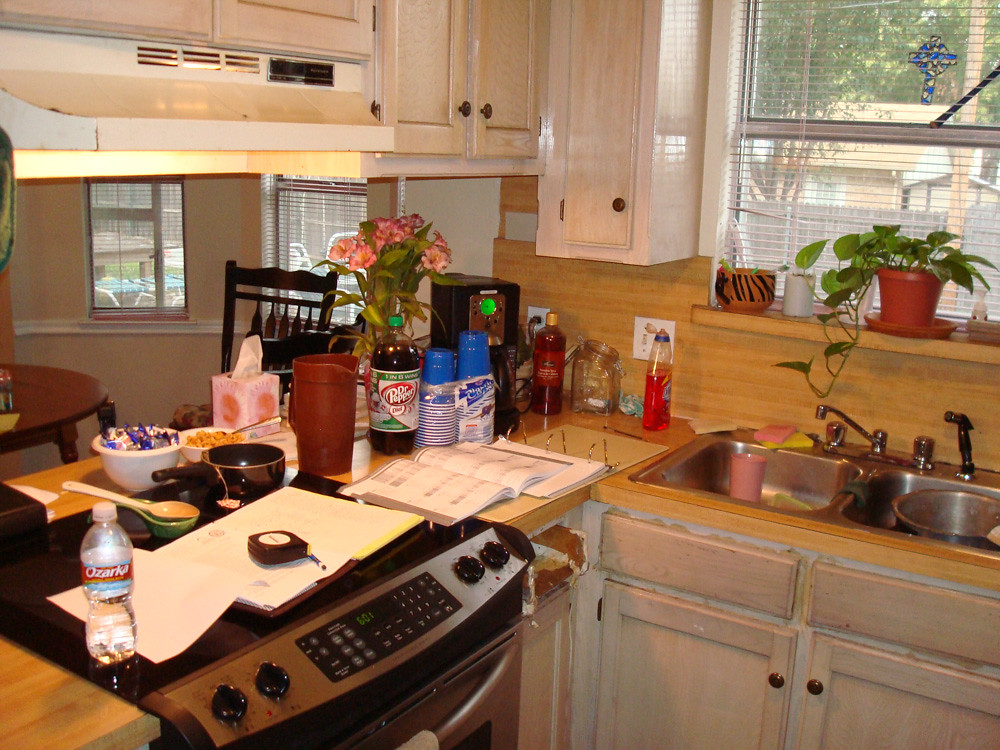The image depicts a cozy and well-organized kitchen primarily situated on the right-hand side. At the center of the scene is a gleaming stainless steel sink, which reflects the ambient lighting. Below the sink are neatly arranged cupboards, likely housing essential kitchen utilities. Above the sink, a window provides a picturesque view into the outside world. On the windowsill sits a vibrant green plant in a dark tan-colored pot, accompanied by a matching plate underneath to catch excess water and protect the wooden sill.

Alongside the plant, the windowsill hosts a collection of miscellaneous items, including a small white figurine, a white cylindrical container, and another decorative pot adorned with black, slightly left-leaning vertical lines. A white shade covers the window, lending a gentle diffused light to the scene. Prominently featured on the window is a striking translucent cross, adorned with varied shades of blue and bordered by a black outline, which suggests materials such as plastic or glass.

To the left of the sink, the cabinetry continues with a combination of very tall and shorter double-doored cupboards, providing ample storage space. Above the stove is a functional hood, with two covers designed to efficiently vent steam. The stove itself features a glass top and likely four burners, situated above an oven compartment ideal for baking. Surrounding the stove is a varnished and sealed wooden countertop, cluttered with various kitchen items.

Beyond the stove, the scene extends into an adjacent room, where dark-stained chairs and a varnished table can be seen. This room is lit by two windows draped with white shades. Additionally, the sink contains some items, indicating ongoing or recent use. To the right of the stove, a vase of fresh flowers, predominantly pink with white centers and complemented by green foliage, adds a touch of natural beauty to the space.